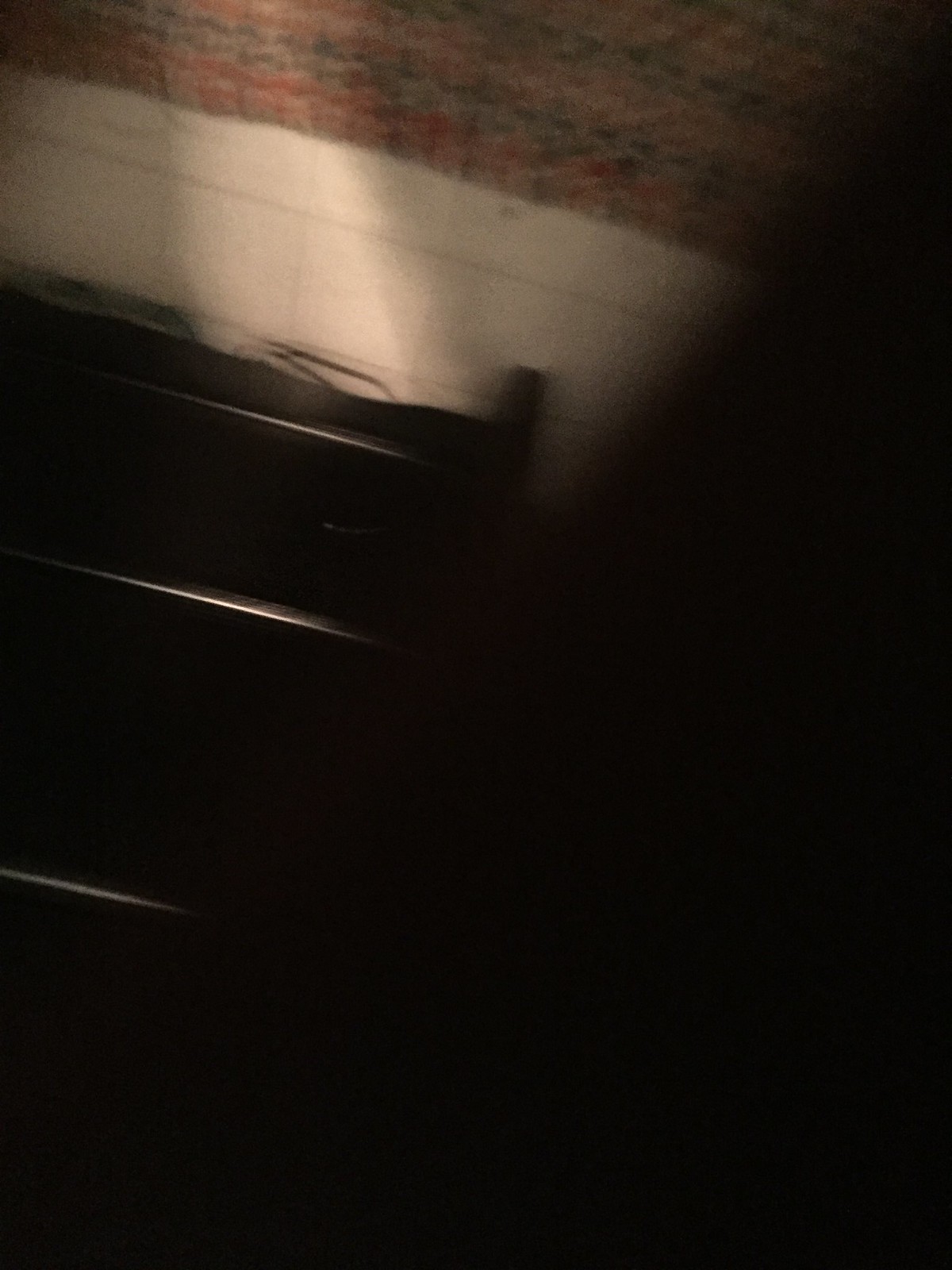This image appears to be an accidental photograph, possibly taken while someone was putting their phone away. Over half of the picture is completely dark. In the upper third, there is a white tiled floor with black lines, and a colorful, striped rug lying horizontally across it. This part of the image is illuminated, with light coming from below, creating shadows on either side. There's an upside-down stand or piece of furniture with several shelves and possibly a cord coming from the bottom, situated in the background. The stand's legs are facing the top of the screen. Additionally, there is a black shadow extending from the bottom right to the center left, adding to the overall darkness of the image.